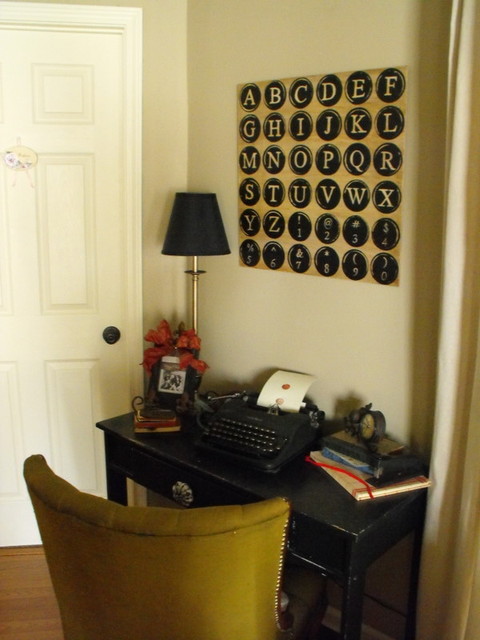A vertically rectangular, full-color photograph taken indoors, likely staged, shows a small, cozy corner of someone's home. On the right-hand side, the edges of a white curtain are visible, while on the left, a closed white door with a black handle stands out. Central to the image is an old-looking black wooden desk with a black typewriter that has a piece of white paper inserted. The desk also holds a couple of books and a black lamp with a gold-colored pole. A yellow-green high-back chair is positioned in front of the desk. Above the desk, a unique piece of artwork featuring the alphabet and numbers from 1 to 0 is displayed on the wall. The artwork, resembling typewriter key impressions with black circles on a gold or copper background, adds a vintage touch to the setting. A few red flowers are also visible on the left side of the table, adding a hint of color to the scene.